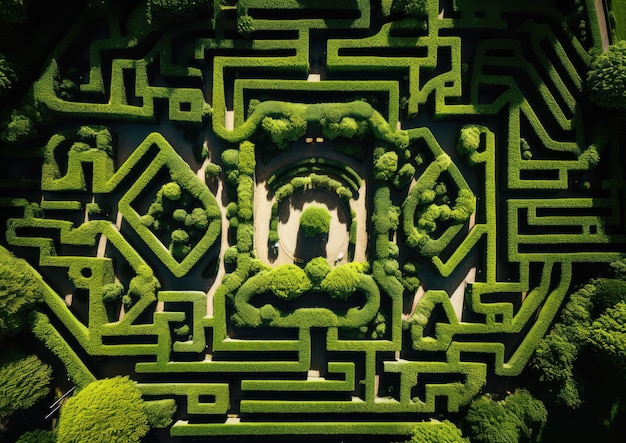This image presents an aerial view of a meticulously designed and well-manicured maze, sculpted from tall, verdant hedges. At the heart of the labyrinth, which is centrally featured in the image, lies a distinct middle area highlighted by a small, round plant or tree, encircled by a semicircle of smaller bushes. Surrounding this central decoration, the hedges form a square pattern. This central section is further enclosed by a diamond-like design created by the meticulously pruned pathways of the maze.

From the top perspective, the intricate pathways of the maze weave in all directions, forming a complex network of trails. The ground beneath the hedges exhibits a peach color, providing a striking contrast to the lush green foliage. Flanking the maze on both sides are towering, dense trees that form a natural boundary, appearing particularly prominent on the left and right edges of the image. Towards the bottom left and bottom right corners, larger trees or bushes dominate the view, obscuring portions of the maze beneath. This seamless blend of natural elements and geometric design creates a visually captivating garden area, combining the orderly aesthetics of horticultural art with the natural beauty of the surrounding landscape.